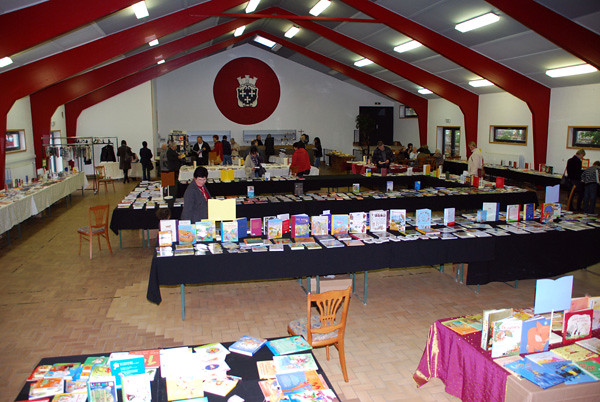This photo captures the interior of a large, light-colored meeting hall, possibly a church, hosting an event that appears to be a book or craft fair. The room is characterized by its open span ceiling with red beams and fluorescent lights. Dominating the back wall is a large red shield-like insignia featuring a face with a crown and crosses for eyes and a mouth. The floor is patterned with orangish-tannish tiles resembling bricks.

In the foreground, a variety of tables, some with black or pink tablecloths, are laden with books. One table in the bottom left corner is short and black, covered with books lying flat. In contrast, the table in the bottom right corner, adorned with a pink tablecloth, has books both lying down and stacked upright. Farther back, a long table holds numerous books, with several standing upright to attract attention. On the sides of the hall, tables against the walls are also heaped with books and various objects, some covered with white tablecloths.

A brown wooden chair with a high back is positioned in the near portion of the room, and several other chairs are scattered around the tables. The scene is bustling with people, especially concentrated toward the back under the large red insignia. Notably, a woman in a red shirt and gray blazer stands out in the foreground. Overall, the space feels vibrant and busy, with an almost endless array of books and items available, suggesting a thriving indoor fair atmosphere.